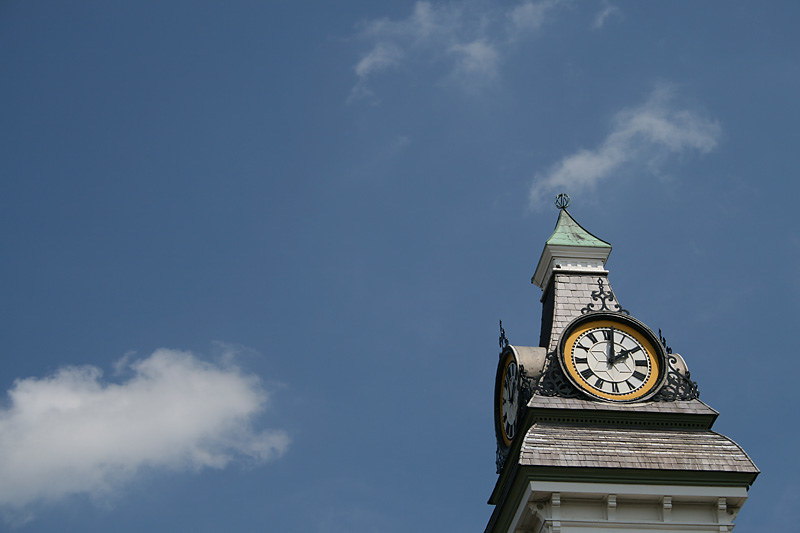In the image, you see the top section of a clock tower, possibly part of a church or cathedral, characterized by a prominent, pointed, shingled roof covered in gray and green tiles. The structure has a distinctly castle-like appearance with triangular, pointed tops. The tower features large, circular clocks set on multiple sides, with two clearly visible. Each clock is framed in dark metal housing, with an orange outer rim. The clock faces are black and white, with Roman numerals marking the hours. The longer hand points to 12, while the shorter one points to 2. The scene is set against a bright, clear blue sky, with a few wispy clouds scattered in the background.